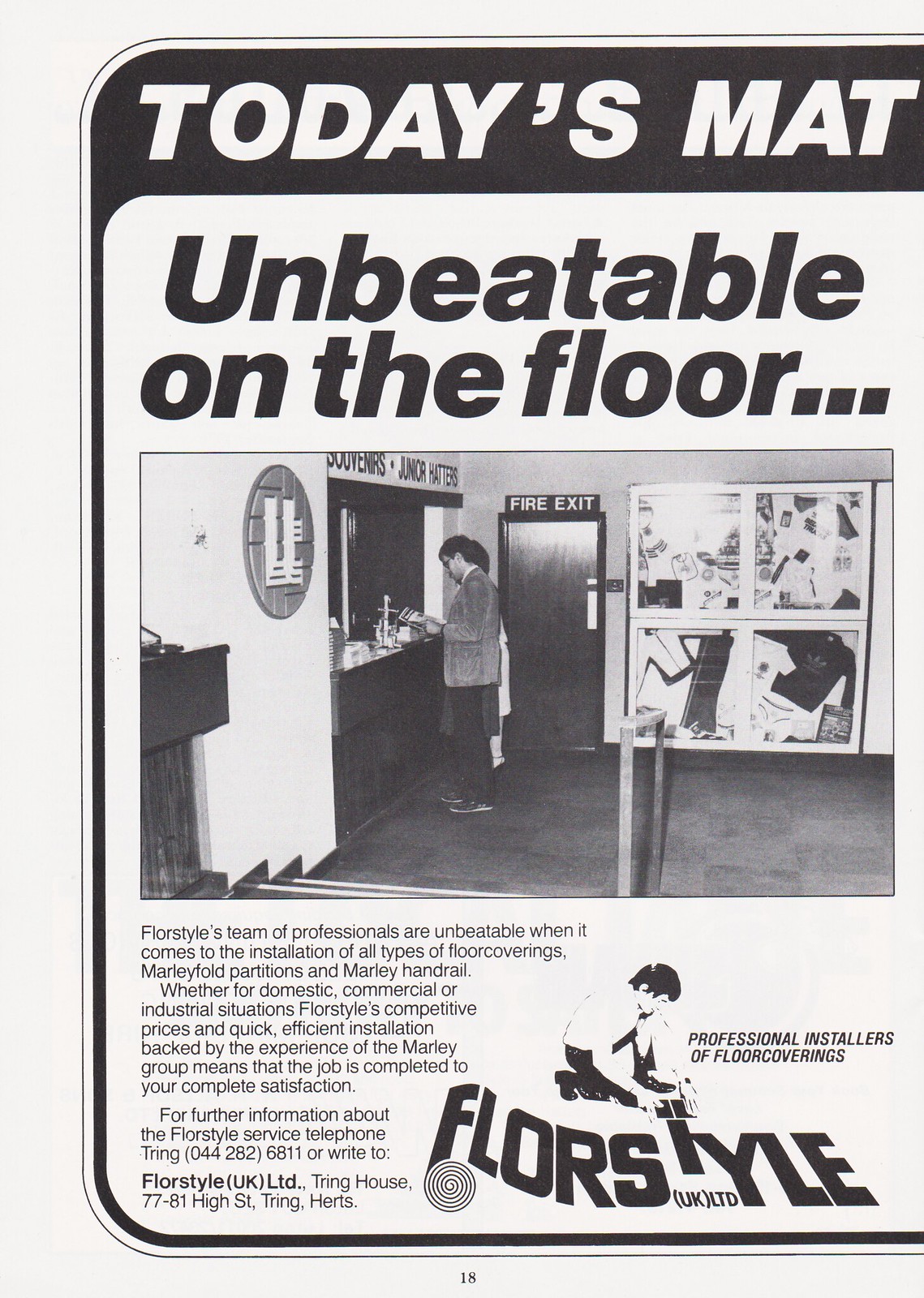The image prominently features an old black-and-white advertisement, centered within the frame, analogous to an old poster or booklet page capturing the entire photo. The advertisement's design includes rounded corners on its top and left, with the right side slightly cut off. The text at the top, incomplete due to the cutoff, reads: "Today's M-A-T, unbeatable on the floor..." followed by a detailed promotional message. The central part of the advertisement features a picture of two individuals standing at an open counter, with a visible fire exit door in the background and a secondary poster to the right, suggesting the scene is set in a lobby. The ad extensively describes FloorStyle's professional services, highlighting their expertise in the installation of various floor coverings, including Marley fold partitions and handrails, suitable for domestic, commercial, or industrial settings. It emphasizes their competitive pricing and efficient installation, backed by the Marley group's extensive experience to ensure customer satisfaction. Beneath the ad, contact information is provided: "For further information about FloorStyle service, telephone Tring 044-282-6811 or write to FloorStyle UK Ltd, Tring House, 77-81 Hyde Street, Tring, Hertz." The color palette of the image is predominantly shades of white, black, and gray, enhancing its vintage feel. The text also mentions "professional installers of floor coverings," encapsulating the core theme of this nostalgic advertisement.